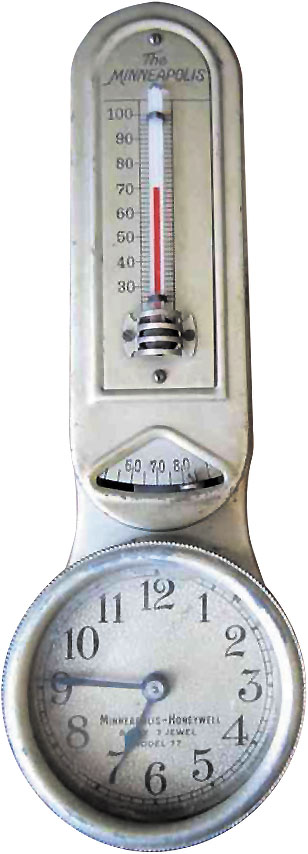This image features a unique antique combination of a clock and a thermometer. The base of the piece is reminiscent of a wide-handled spoon, crafted in an antique silver finish. At the bottom, the circular clockface displays black numerals with the current time set to 6:46. 

Directly above the clock, forming the handle of the spoon-like shape, is the thermometer. The thermometer scale appears to start at 30 and goes up to 100, indicating the temperature. At the very top, it is labeled "Minneapolis." The current temperature reads approximately 69°F. 

In the middle section of the thermometer, there are additional markings ranging from 60 to 80, which seem to serve a special function, potentially allowing the user to set a desired temperature.